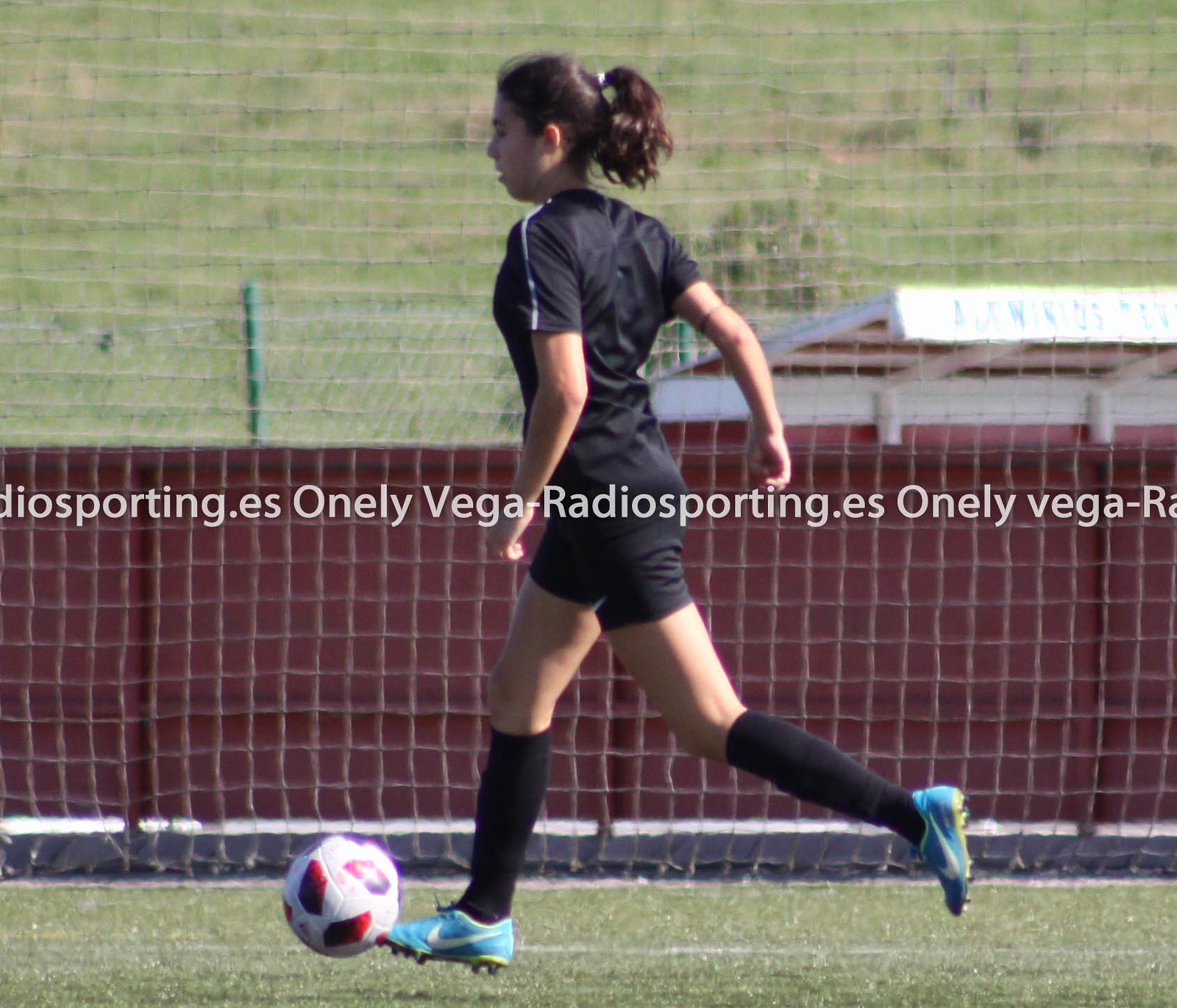The image captures a young girl, likely a soccer player, in action on a green soccer field. She is wearing an all-black outfit consisting of a uniform top, shorts, and knee-high socks, complemented by her blue Nike cleats. Her dark brown hair is tied back in a ponytail. Positioned prominently in the image, she is running towards the left, focused on kicking a red and white soccer ball in front of her. The background includes a mix of elements: immediately behind her is a netting, possibly part of a goal, followed by a maroon or red wall. To the right, a bush and an awning are visible, while a green pole can be seen on the left side of the image. The field itself features green grass and a visible white line. Superimposed across the middle of the image, in a horizontal line, are repeated watermarks with the text "dosporting.es," "onlyvega," and "radiosporting.es." The vivid colors and dynamic posture of the girl create a vibrant and engaging scene.